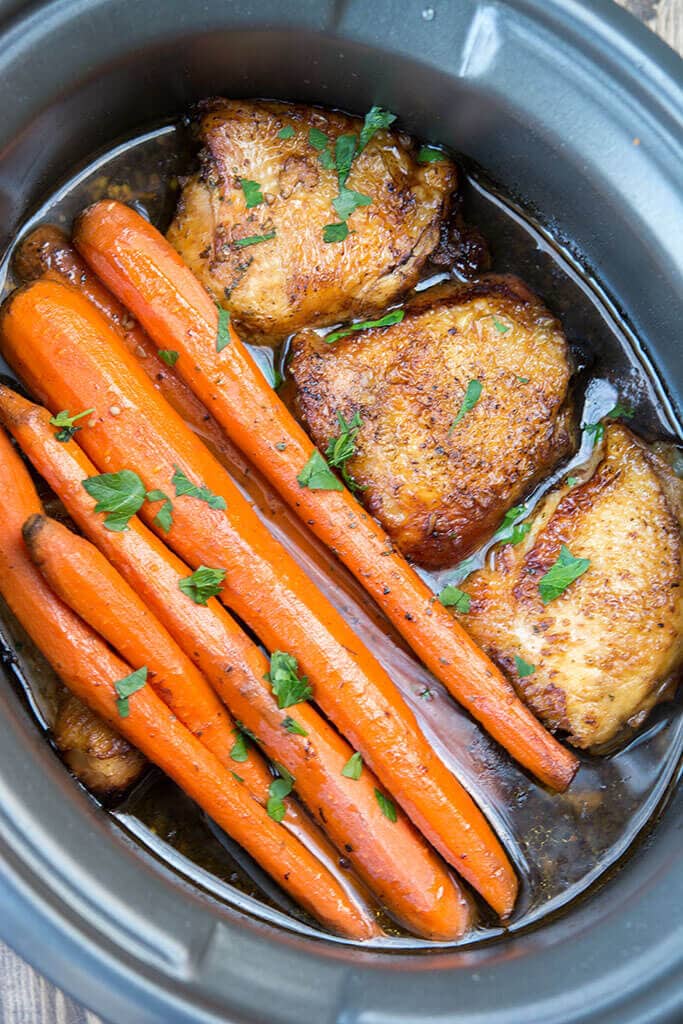This image captures the view inside a gray, oval-shaped crock pot with a shiny finish. The interior of the pot is black and contains a layer of dark, glistening liquid. On one side of the pot, a cluster of whole, peeled carrots is arranged, their bright orange hue contrasting starkly with the dark liquid around them. The carrots are generously topped with chopped parsley. Adjacent to the carrots are three browned and golden pieces of chicken, likely chicken thighs, which appear well-seasoned and may have a light breading. The chicken pieces are placed in the liquid, with additional chopped herbs, possibly basil, sprinkled over them. The composition of the crock pot contents showcases a hearty, rustic dish in progress.